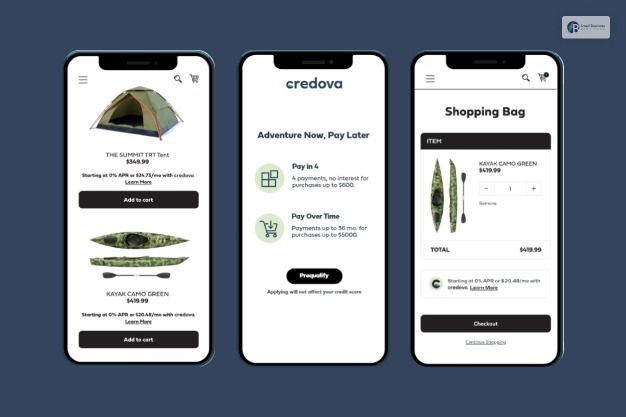This composite image features three separate smartphone screens side-by-side against a dark grayish background, each displaying different shopping-related content. 

1. **Left Phone Screen:**
   - Displays an online shopping page showcasing two products.
   - The top product is a "Summit TRT tent" priced at $349.99, accompanied by an "Add to Cart" button. Additional text details are present but too small to read.
   - Below the tent, there is a "Camo Green Kayak" priced at $439.99, illustrated with multiple images showing the kayak from above, from the side, and with a paddle. This also includes an "Add to Cart" button.

2. **Middle Phone Screen:**
   - Displays a promotional page from "Cordova" with the headline text "Adventure Now, Pay Later."
   - Features two circular icons: the first contains four squares and states "Pay in Four," while the second has a shopping cart and an arrow, stating "Pay Over Time." Both icons are accompanied by text that is too small to discern.
   - The bottom section of this screen has a black button with unclear text, likely saying "Pre-qualify," followed by another line of small black text.

3. **Right Phone Screen:**
   - Shows a shopping cart page with the title "Shopping Bag."
   - The principal item listed is the "Camo Green Kayak."
   - Includes a couple of small text lines near the bottom, which are indistinct.
   - Features a prominent black "Checkout" button at the bottom.

In the upper right corner of the overall image, there is a small rectangular gray box containing an unreadable circular logo and text.

This detailed description aims to capture the key elements and layout of the composite image for clarity.